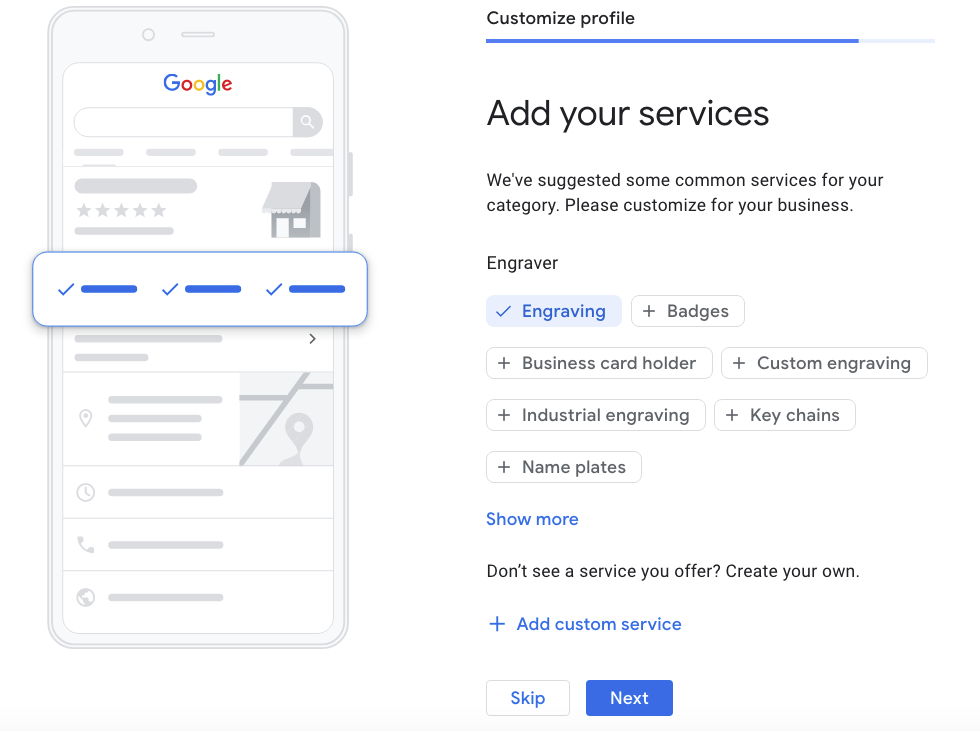On the right side of the interface, there is an option labeled "Customize Profile" in black text, with a blue line beneath it that gradually transitions to a lighter shade as it extends to the right. Below this option, another section invites users to "Add Your Services," highlighted in black text. It includes a prompt that reads, "We've suggested some common services for your category. Please customize for your business."

In this segment, various service options are listed in black text, with some accompanied by specific visual indicators:
- "Engraver" is followed by a blue rectangle containing the word "Engraving" along with a checkmark.
- The word "Badges" features a plus sign beside it. 
- Additional listed services include "Business Cardholder,” "Custom Engraving," "Industrial Engraving," "Keychains," and "Nameplates."

Below these options, "Show More" appears in blue text, followed by a prompt in black text: "Don't See a Service You Offer? Create Your Own," alongside a blue plus sign labeled "Add Custom Service." Users can also choose to skip this step, or proceed by clicking the "Next" button in a blue rectangle.

To the right of this interactive area, the word "Google" is displayed next to an image of a cell phone.